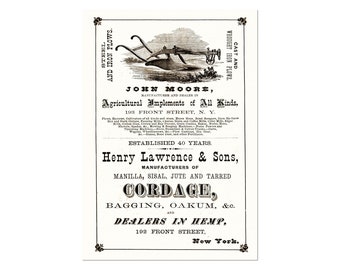The poster is an old-fashioned, black-and-white advertisement resembling early printing styles, set against a white background. Dominating the poster is the name "John Moore," with a headline that reads "John Moore Agricultural Implements of All Kinds." A finely detailed illustration at the top depicts farming equipment or possibly a plant, rendered in black and brown hues. The text, while abundant and small, prominently features various business details: "Established 40 Years," "Henry Lawrence & Sons, Manufacturers of Manila, Sisal, Jute, and Tarred Cordage, Bagging, Oakum," and also mentions they are "Dealers in Hemp." The address "192 Front Street, New York" appears twice, suggesting a clear location for the business. Despite the richness in information, much of the text remains challenging to read due to its diminutive size.